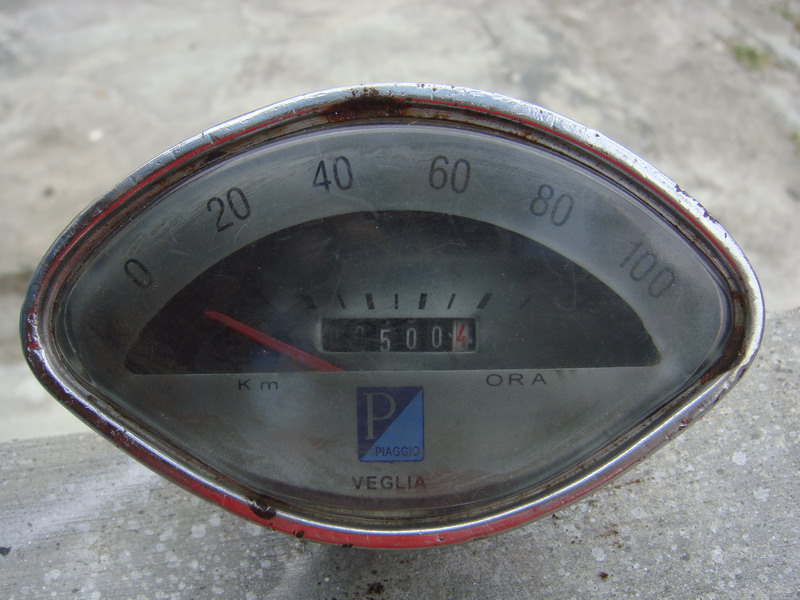This photograph captures an oval-shaped odometer, designed to measure the distance traveled by a vehicle, prominently displayed on a gray, concrete surface. The odometer features an indicator needle, often referred to as a "red stick," which points to the number of kilometers traveled. The scale on the odometer progresses in increments of 20, ranging from 0 to 100, as you read from left to right. The current reading shows 5004 kilometers, with the first three digits (500) in white and the last digit (4) in red.

The odometer has an outer design comprising both silver and red outlines, contributing to its distinctive appearance. Additionally, the brand name "Piaggio" is prominently displayed on the device, with the "P" emblem set within a blue rectangle. This odometer combines practical functionality with a visually appealing design, making it an eye-catching feature on the concrete backdrop.